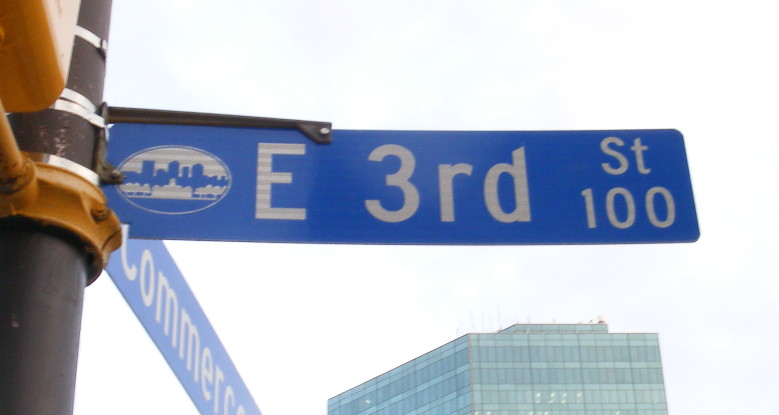The image captures a close-up of a street sign at the intersection of East 3rd Street and another street that appears to be Commerce, though the latter is partially obscured. The blue street signs are affixed to a brown metal pole with orange fittings, likely for a traffic light or street signal. The primary sign, prominently displayed from left to right, reads "E 3rd Street 100" and features an oval emblem of a cityscape to the left of the "E." A second, downward-facing sign, partially visible behind the pole, seems to read "Commerce." The scene suggests an American city, characterized by these specific street signs and urban infrastructure.

In the background, a tall commercial building with a glass facade is visible, suggesting a downtown area. The building, likely an office structure, has multiple floors with numerous windows. Above and around the structure, the sky appears white, providing a stark backdrop. The overall photograph is detailed, focusing on both the street signs and the architectural elements indicative of a bustling urban environment.